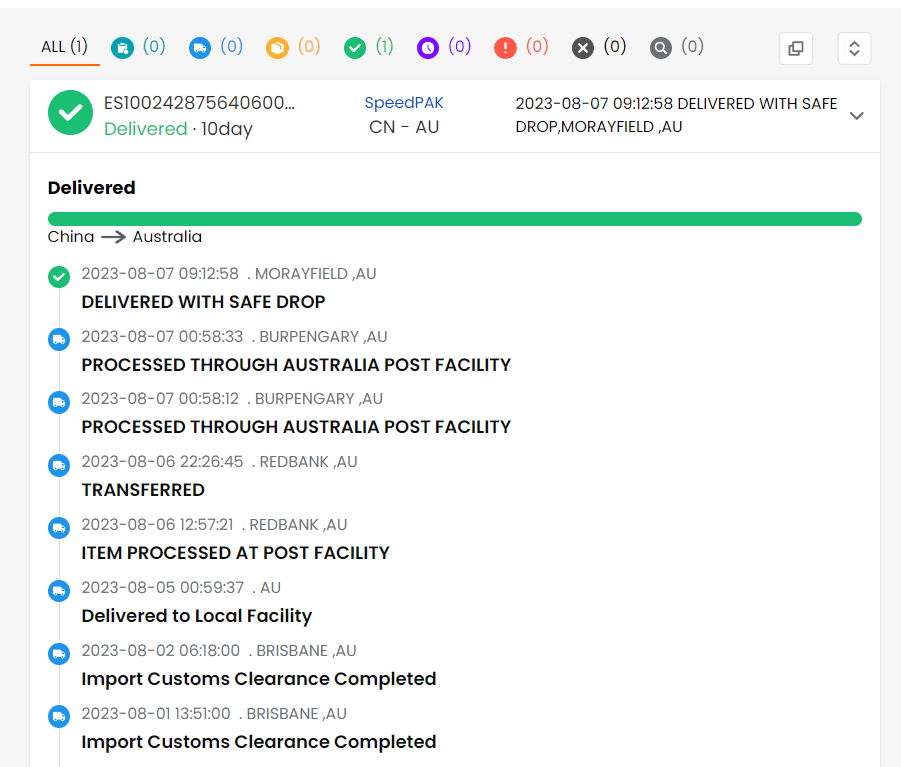The image features a detailed tracking timeline for a package delivery from China to Australia. 

At the top of the image, a gray background provides contrast for a series of circles and connecting lines, each accompanied by corresponding text. The first section begins with a black bar that reads "(1)," followed by a red line. Adjacent to this, a series of colored circles with corresponding labels in parentheses are displayed: 

- A blue circle labeled "(0)"
- An orange circle labeled "(0)"
- A green circle labeled "(1)"
- A purple circle labeled "(0)"
- A pink circle labeled "(0)"
- A dark gray circle labeled "(0)"
- A light gray circle labeled "(0)"

Below this sequence, text indicates various stages of the delivery process:

- "Delivered" in green text
- "10-day" in black
- "Speed pack" in blue
- "CN-AU" in black
- Dates and timestamps: "2003-08-07" and "09:12:58"
- "Delivered with safe drop, Moiré Field, AU"

A thin gray line traverses across the image with bold black text stating "Delivered," below which is a thicker green line.

The next section elaborates further on the delivery route and stages:

- "China" in black, with an arrow pointing towards "Australia"

Below this, several other lines annotated with dates, times, and locations map the journey of the package:

- A green circle indicates the time "2003-08-07-09-12-58" and location "Moiré Field, AU"
- The package was "Delivered with safe drop"
- It was subsequently processed at an "Australia Post Facility"
- Transferred and processed at another post facility, with further steps including "Delivered to local facility" and "Import customs clearance completed."

Overall, the image meticulously details each step and status update in the package's journey from sender to recipient, highlighting the various processing stages and timestamps associated with its delivery.